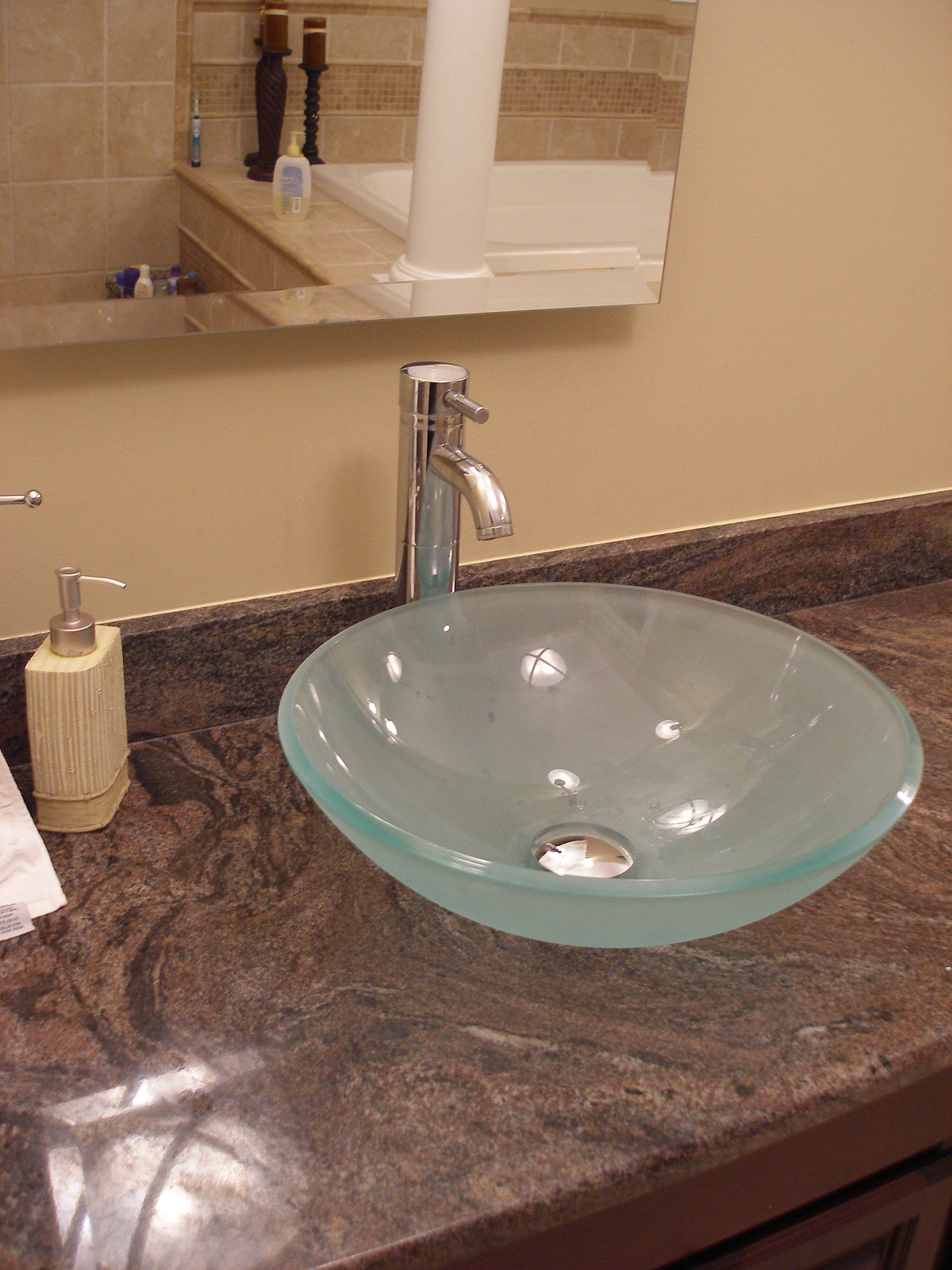This image showcases a sophisticated bathroom setup featuring a distinctive bowl sink made out of blue-tinted, clear glass. The glass bowl sits prominently atop a cultured marble countertop, colored in a rich brown hue. A sleek, single-handled faucet accompanies the sink. To the left of the sink is a yellow ceramic soap dispenser equipped with a stylish silver spout. In the background, through a clean, beveled mirror reminiscent of one you might find on a medicine cabinet, a section of the bathroom with brown tiled columns is visible, potentially adorned with candles. The bottom left corner of the image catches a glare from the overhead light, adding subtle warmth to the scene.